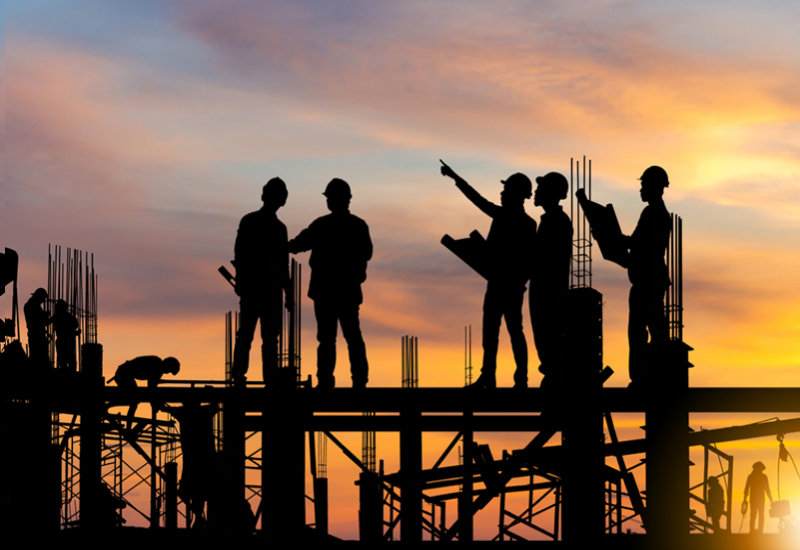In this captivating sunset photograph, a group of construction workers is silhouetted against a vibrant evening sky, awash with hues of yellow, purple, and blue. The focal point is a steel beam where five men stand prominently in the foreground, possibly architects or crew leaders, as indicated by the maps they hold and the way they are pointing upwards. The central figure, likely the foreman, gestures with his right hand while clutching a scroll in the other, directing the team's attention. Beside him, another man also holds a scroll, contributing to the air of coordination and planning that pervades the scene.

In the background, a mix of shadowy figures can be seen diligently working. To the back left, another group of men crouches, intent on their tasks, while to the right, two workers stand on a lower platform beside an elevator, lifting materials. The photograph captures their black outlines against the setting sun's gradient, transitioning from a whitest light in the bottom right corner to a rich orange-yellow hue, melding into the varied colors of the sky above. Additionally, the rebar poking through the cement in places hints at the ongoing progression of this high-rise project, an intense and beautifully captured moment in the realm of construction.